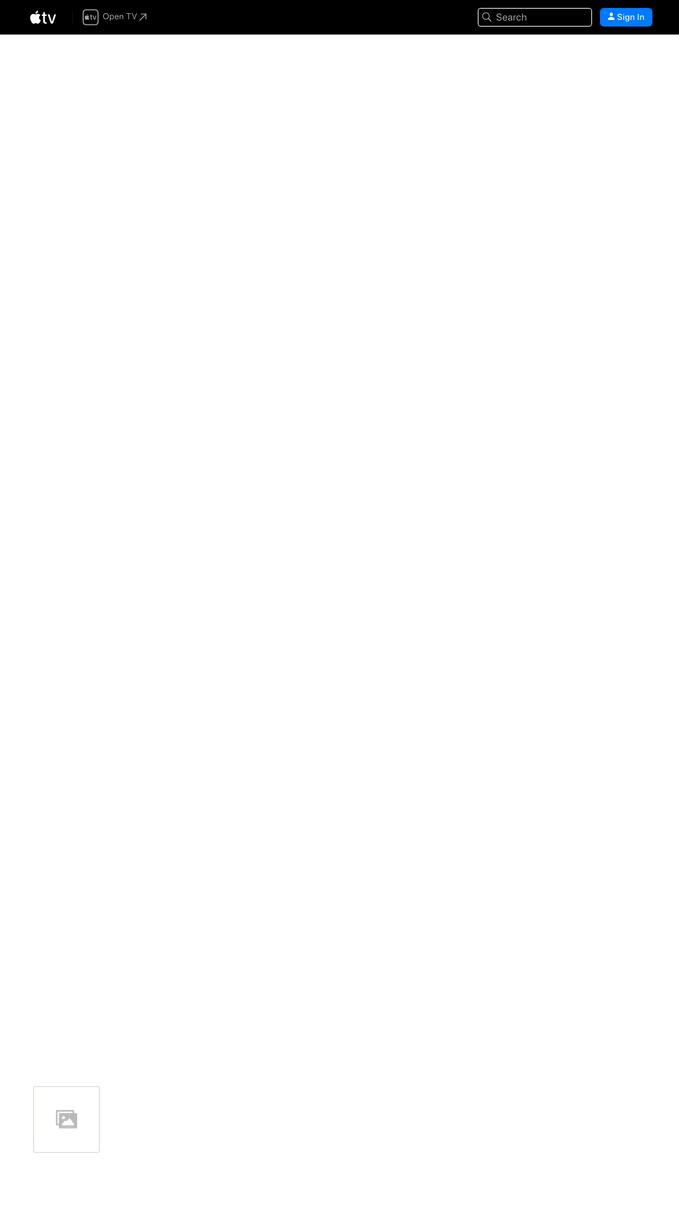The image features a long horizontal rectangle with a black backdrop at the top. On the left side of the rectangle, there is an Apple logo accompanied by the text "TV" in white. Adjacent to this is a small square with rounded corners containing indistinguishable small text. To its right, the words "Open TV" are displayed, along with an arrow pointing upwards and to the right diagonally. Shifting focus to the right side of the rectangle, there is a grey-outlined search bar featuring a magnifying glass icon on the left and the word "Search" in grey, left-aligned within the bar. Further to the right, a blue rectangle with rounded corners contains a white silhouette of a person and the text "Sign In" in white font.

Below this main black rectangle, at the very bottom of the image, a grey square border appears on the left side, followed by significant white space. Centrally located at the very bottom is another grey square, this time with a silhouette of a sun and mountain range inside, representing an image icon.